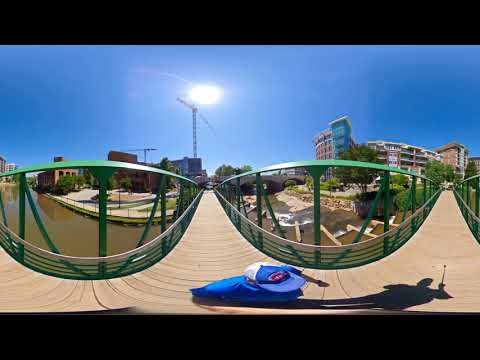The image captures a vibrant 360-degree view from a fisheye lens, showcasing a young man standing on a wooden pedestrian bridge. The bridge features distinct green metal girders and rails, and casts a noticeable shadow of the man holding a selfie stick on the planked surface. He is wearing a blue t-shirt and a blue and white baseball cap with a red logo. Below the bridge, there is a murky body of water with a dock and a few boats. On the horizon, the scenery opens up to a bustling cityscape. To the right, there are several buildings including a prominent four or five-story structure, possibly a hotel with a parking garage. Additionally, a rounded edge building, perhaps made of brick, and a blue tower can be seen in the distance. On the left, several buildings probably used as apartments dot the landscape. The blue sky above is clear, illuminated by the sun, and features a couple of cranes suggesting ongoing construction in the area. The scene is devoid of other people and text, culminating in a tranquil yet dynamic urban snapshot.